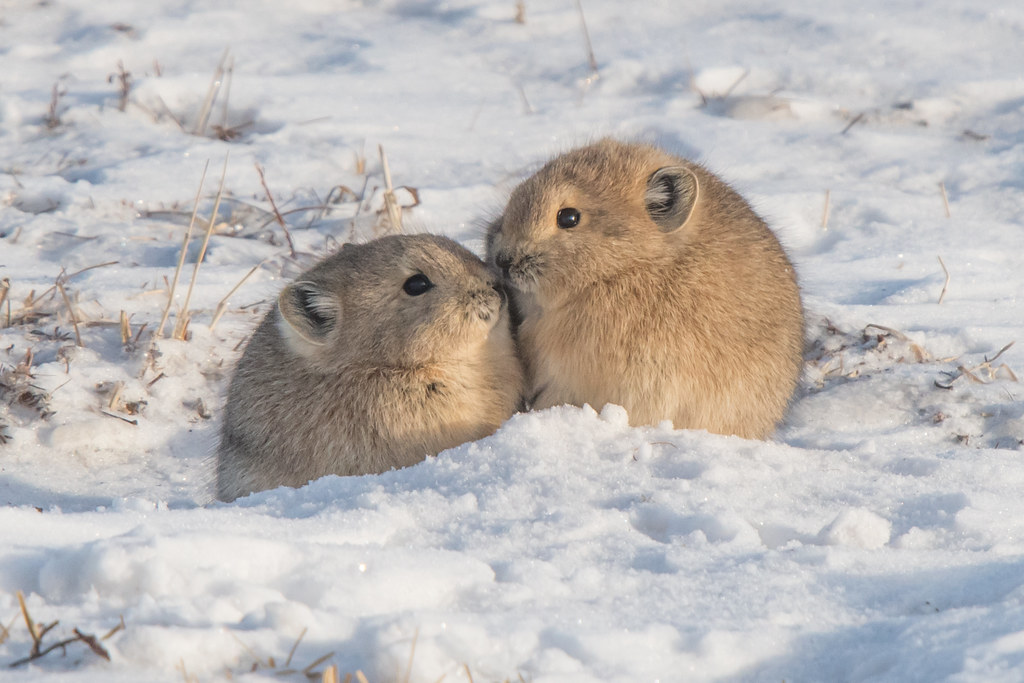This is a horizontally aligned rectangular photograph with no border, capturing a close-up scene in a snowy landscape. The ground is blanketed with white snow, sporadically dotted with blades of dead, wheat-colored grass peeking through. The land appears flat and level. In the center of the image are two round, chubby, furry creatures that resemble guinea pigs or perhaps small pikas. Their light to medium brown fur and tiny, slightly lighter bellies contrast against the bright snow. They have small ears, black bead-like eyes, and nearly touch noses, almost as if they're kissing. Their bodies are round and puffed up as they sit huddled together, with the snow covering their feet and part of their lower bodies. The sunlight reflecting off the snow enhances the serene and adorable nature of the scene, with the two animals as the clear focal point amidst the otherwise sparse and snowy background.